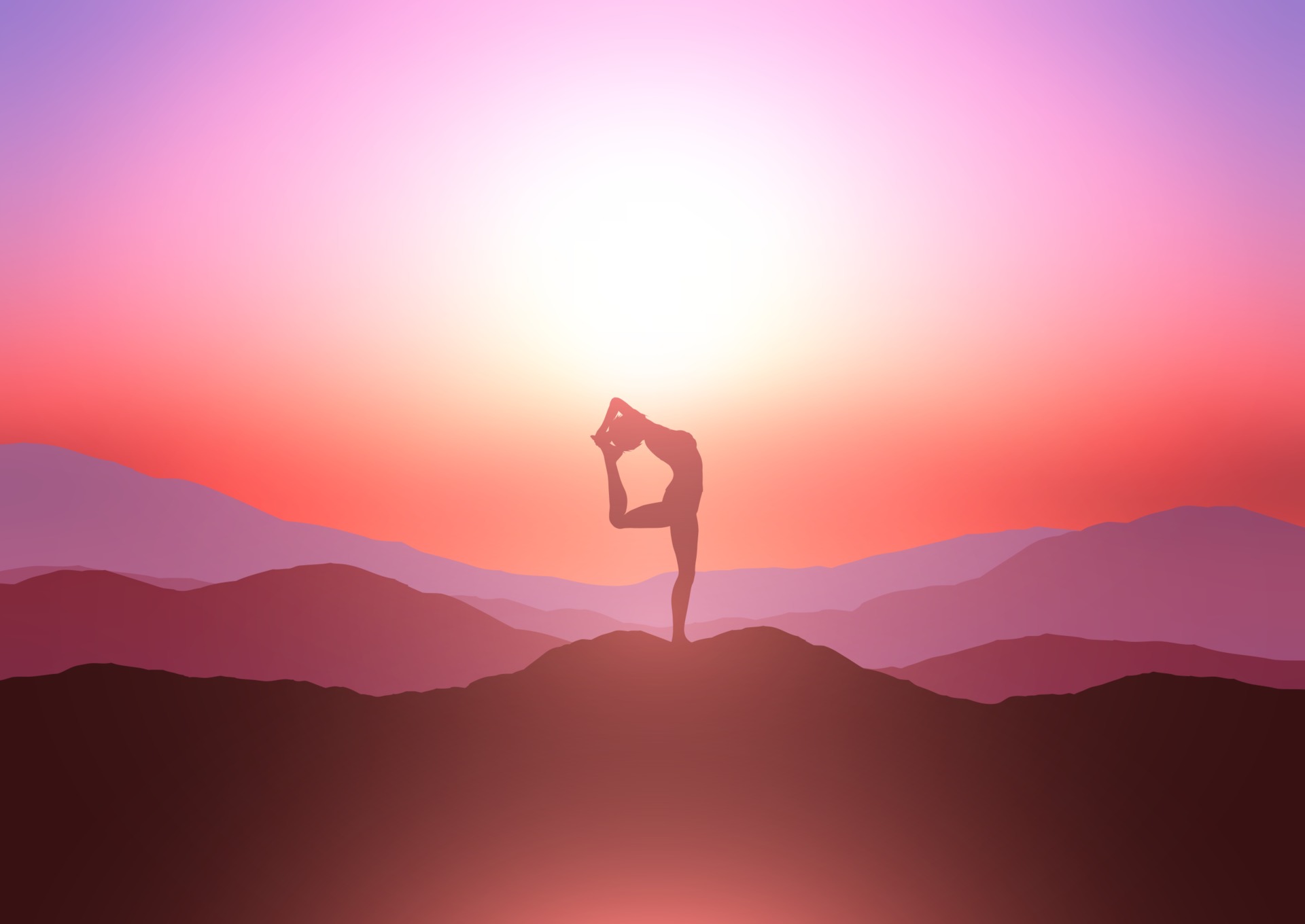The image depicts an inspiring, highly stylized scene of a woman striking a yoga pose at the summit of a series of mountains during what appears to be a sunset or sunrise. The dominant hues of the image transition from dark red to mauve to various shades of purple and violet, culminating in an orange sky with a central yellowish glow, suggesting the presence of the sun. In the foreground, the silhouette of the woman is prominently featured. She stands on her left leg with her right leg bent backward at a right angle, lifting her foot to meet her hands while leaning back into a graceful stretch. This pose, involving intricate balance and flexibility, is executed atop a dark red hill, with progressively lighter mountain ridges extending into the background. The entire composition, with its blend of dramatic landscape and delicate human form, exudes an artistic and motivational aura.